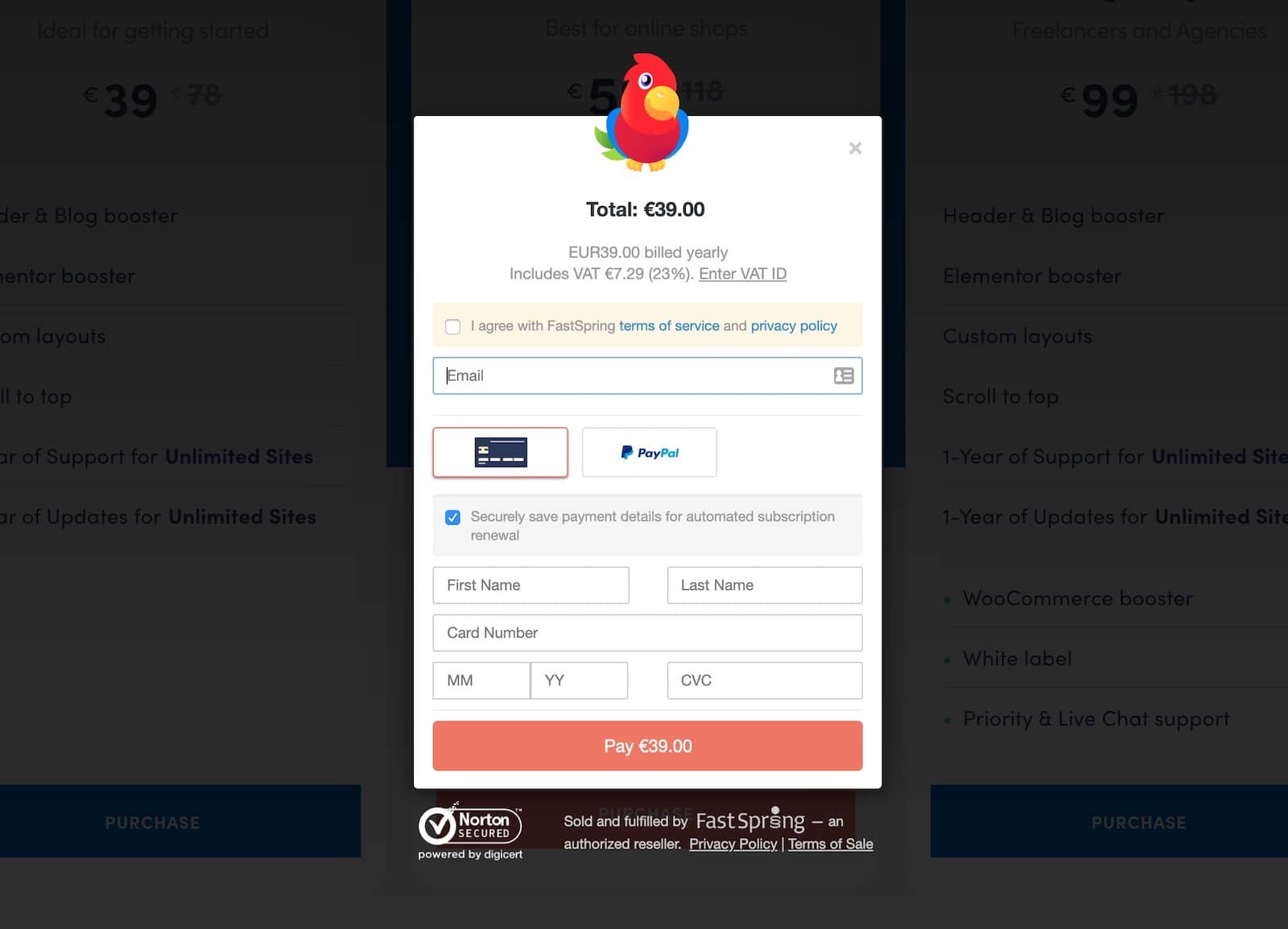The image captures a pop-up window on a website meant for finalizing an order with payment details. The pop-up window is predominantly white and features a cartoonish parrot located at the top center. The total amount due is prominently displayed as "£39.00," indicating the cost of the order. Below this, the text reads "You are billed £39.00 to Gilly" along with a VAT (Value Added Tax) note stating "VAT 23%: £7.29". An instruction to "Enter VAT ID" follows the VAT details.

Lower down the window, there is a checkbox labeled "I agree with Fastbring's terms of service and privacy settings" which users must tick to proceed. A text box is provided for entering an email address. Below this, there are two options for payment methods: one for PayPal and another for credit card payment. The design and layout are clean, user-friendly, and clearly intended to guide the user through the payment process efficiently.